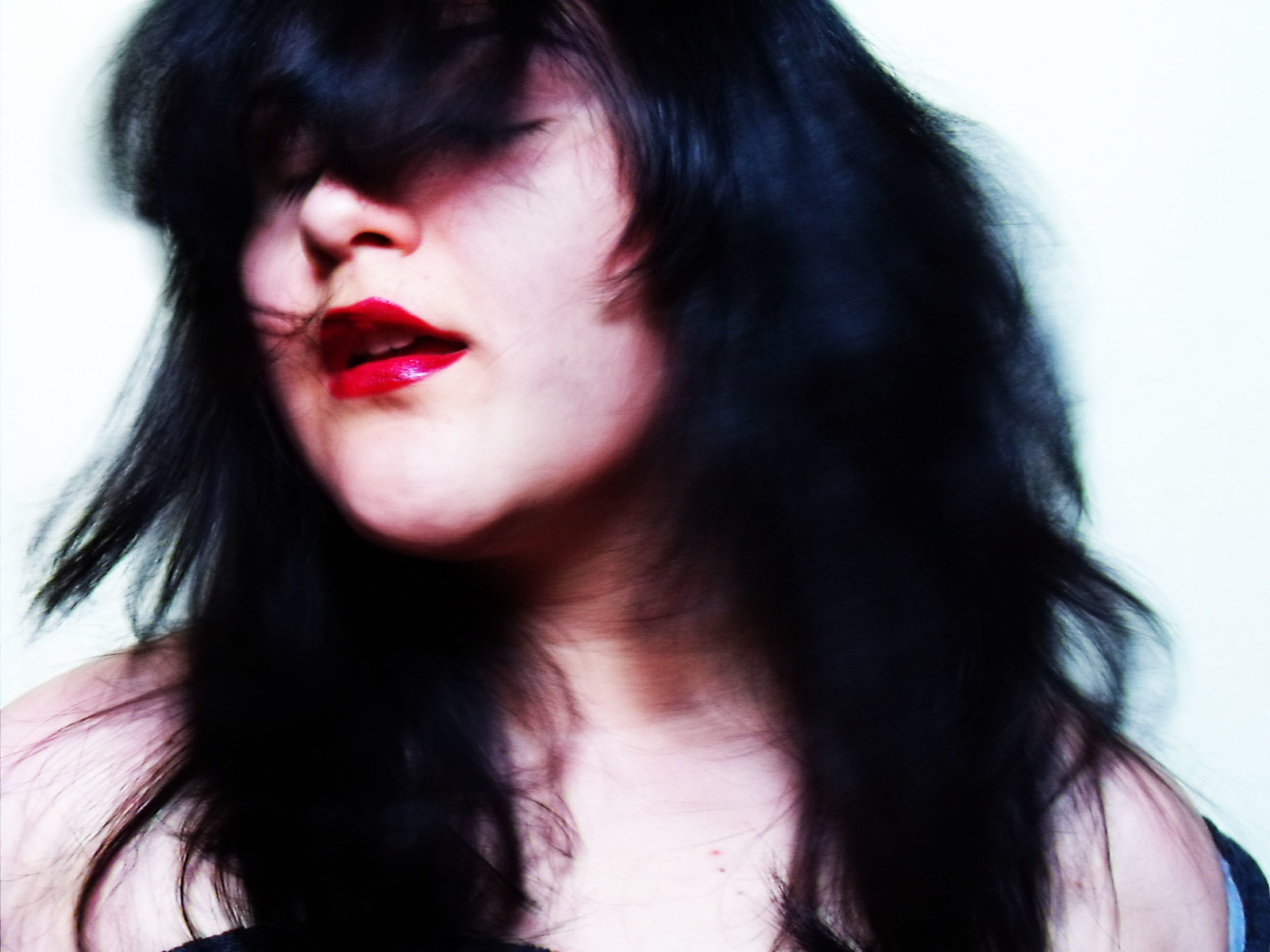The photograph captures a woman in mid-movement, suggested by the blur in her thick, mostly straight but slightly wavy black hair. The shaggy layers and long bangs cover her eyes, with her head angled to the left, emphasizing her red lipstick and slightly open mouth. The top of her head is not visible, only from just above her eyebrows down to her bare shoulders and the upper part of her chest. She appears to be wearing an off-shoulder top, with a glimpse of a blue sleeve visible below her shoulder and a hint of black material near the lower left. The background is predominantly a very light blue, with some darker blue elements on the lower right, set against a white backdrop.